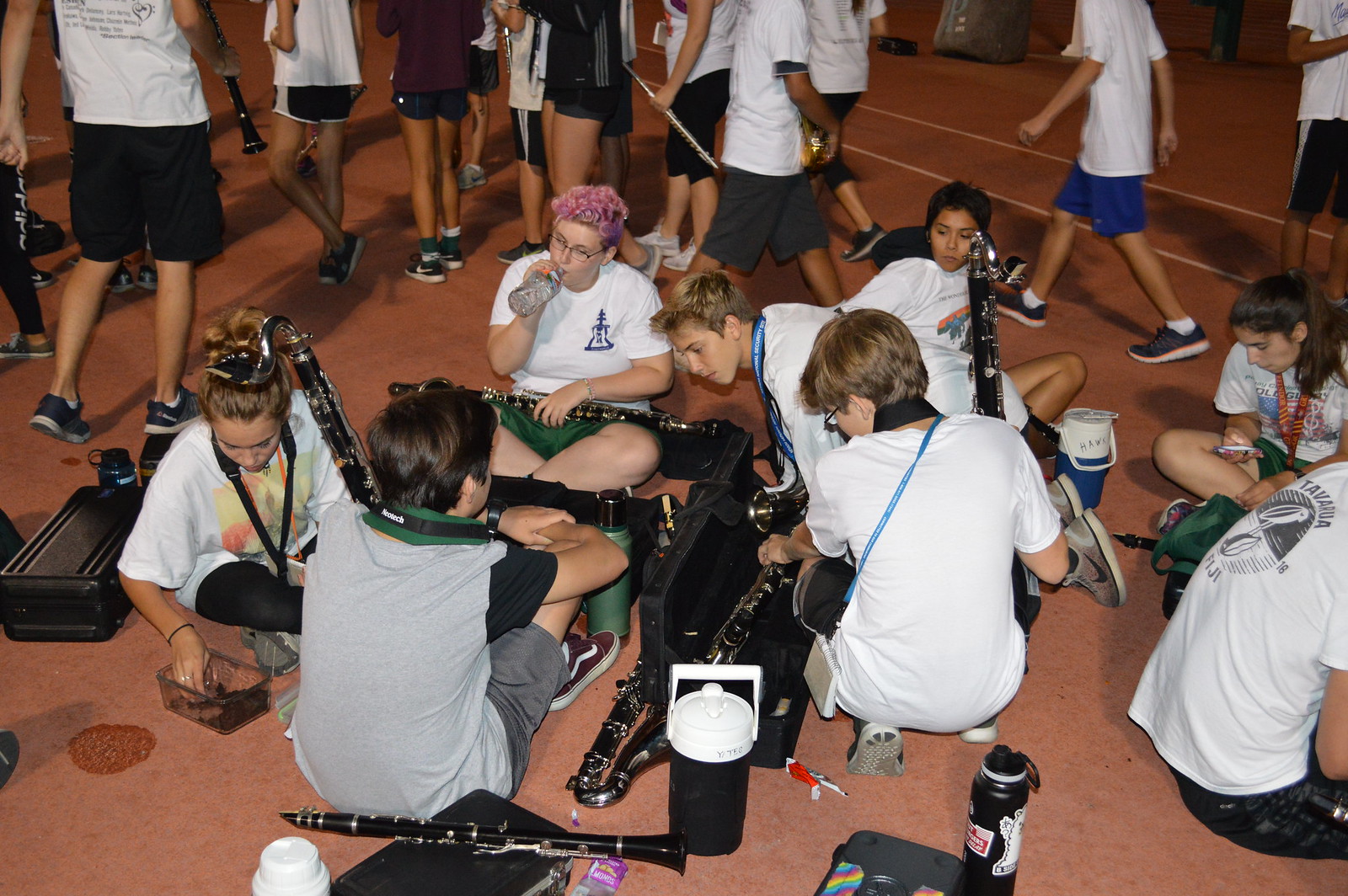In this photograph, we see a group of high school students, casually dressed in white crew-neck t-shirts and shorts, gathered indoors, possibly in an indoor arena, for what appears to be a band practice or a music class. The students are either seated or lying on the ground, with most of them handling various woodwind instruments, predominantly clarinets. Notably, a girl with pinkish hair sits on the left, holding her clarinet in her left hand and a water bottle in her right. Next to her, a boy is hunched over, seemingly inspecting an instrument on the ground. On the far right, a woman is absorbed in her phone, with her clarinet in her lap. The background reveals more students, some standing or walking, and a few others drinking water or just conversing, all contributing to the bustling, preparatory atmosphere of the scene. The floor is scattered with instrument cases, water bottles, and thermoses, indicating a break or a moment of preparation before they commence playing.